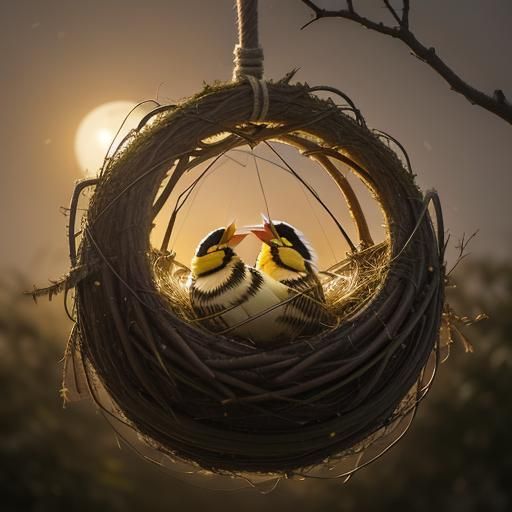The image depicts an impeccably crafted bird's nest, likely AI-generated given its extraordinary perfection and detail. The nest, resembling a finely twisted basket, hangs gracefully from a rope attached to a branch that stretches across the top of the picture. The nest is intricately woven from twigs and straw, appearing almost too perfect to be made by actual birds. Nestled within are two small birds, both with black heads, yellow necks, and orange beaks, facing each other as if communicating or singing, their beaks wide open. Their bodies exhibit vibrant hues—a white body with black stripes for the bird on the left and a bright yellow body with black markings for the one on the right. The background reveals a dusky sky with an ethereal glow, likely from a moon that casts a soft, diffuse light, enhancing the scene's serene and almost surreal beauty. The crisp, photorealistic quality of the image, combined with the lifelike positions and expressions of the birds, further suggests it's an AI-generated masterpiece.